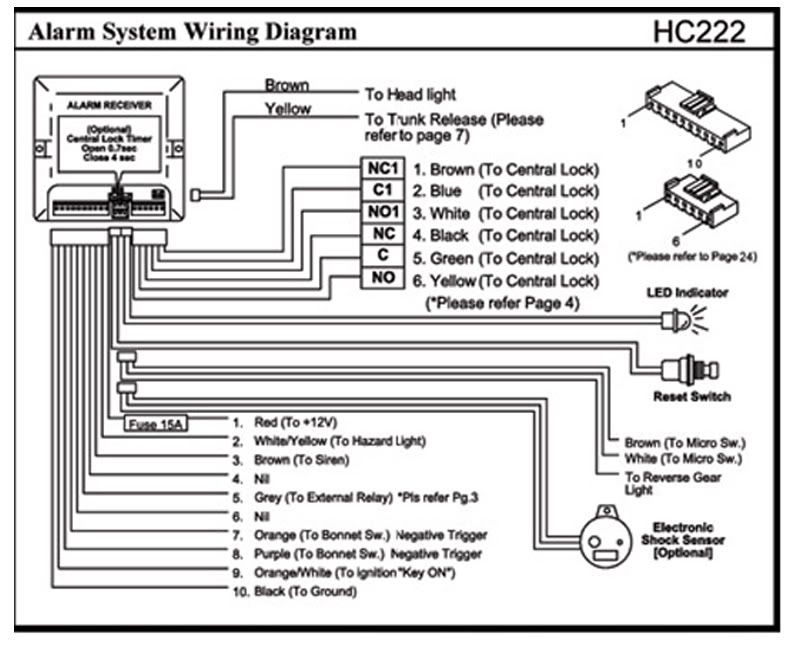The image is a detailed black-and-white schematic labeled "alarm system wiring diagram" in the upper left corner and "HC222" in the upper right corner. Central to the image is a diagram of the alarm receiver, surrounded by a labyrinth of wires denoted by specific colors and labels. The wiring is meticulously organized, with various lines and angles leading to distinct parts and instructional text. Key wires include brown and blue to the central lock, yellow to the headlight and trunk release, and many others connected to the siren, hazard light, and more. The bottom part of the schematic contains numbered connections: red to 12 volts, white and yellow to the hazard light, brown to the siren, and gray to the external relay, among others. Additional highlighted components are an optional electronic shock sensor, an LED indicator, a reset switch, and wires labeled for reverse gear light and ignition key. The presence of terms like "bonnet" suggests the item may be intended for a market outside the United States. Despite the comprehensive information, a barely legible white-on-white watermark suggests ownership of the document.